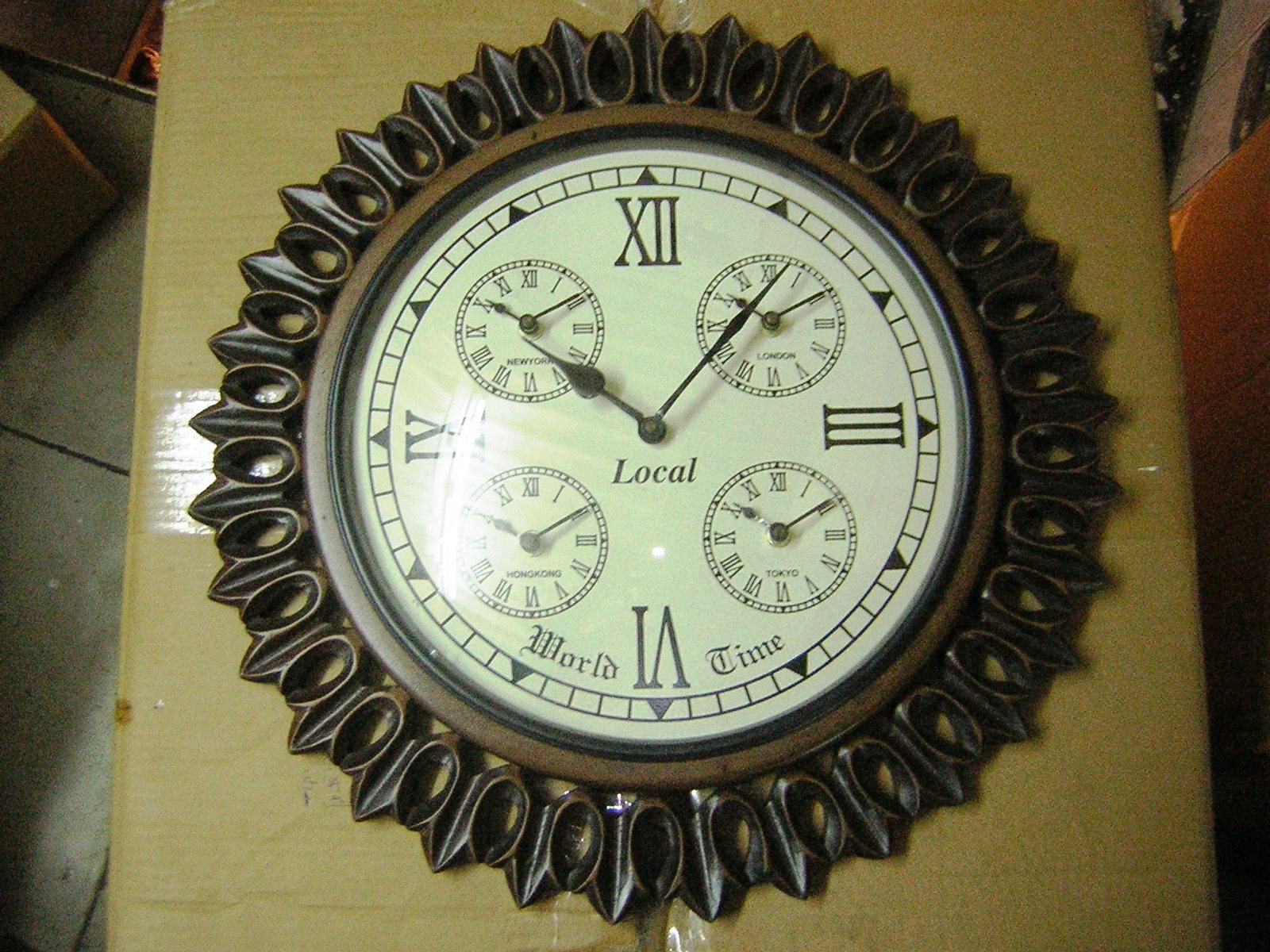The image features a detailed, antique-style clock, prominently placed atop a sealed cardboard box, situated in an ambiguous setting that suggests a workshop or patio. The clock, which occupies about 75% of the photo frame, boasts an ornate rim carved from a deep wooden material with an alternating leaf and possibly acorn pattern. Its frame features a worn brass finish, adding to the antique replica appearance.

The clock face is off-white and covered in glass, reflecting some light. It follows an old-fashioned design with tall, thin Roman numerals exclusively at the 12, 3, 6, and 9 positions. The main clock hands point to 7 minutes past 10, while the central face is complemented by four smaller clocks situated at its corners, designated for London, Tokyo, Hong Kong, and New York. Each of these mini clocks mirrors the larger one in style but includes all 12 Roman numerals.

Under the main hands, the term "Local" is inscribed, while "World Time" is noted below the smaller Hong Kong and Tokyo clocks. The synchronous times displayed on all five clocks suggest they may be battery-operated and currently drained of power. The intricate detailing and meticulously crafted elements of the clock highlight its sophisticated and antique-inspired design.